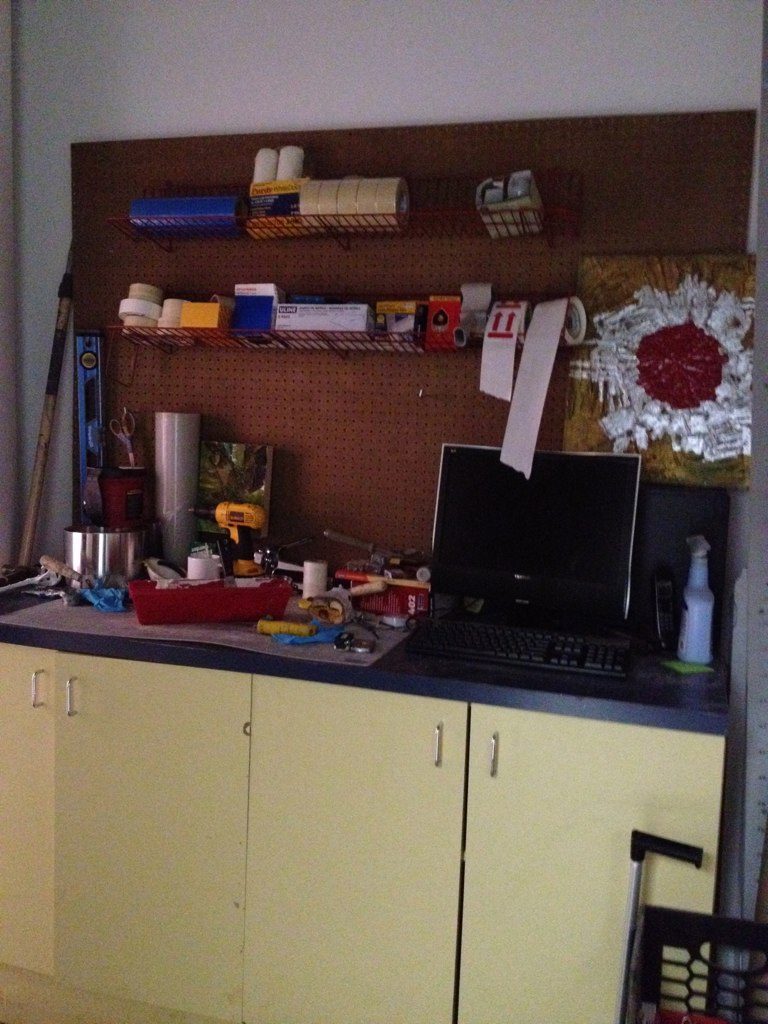The photograph captures a bustling workstation, likely situated in a shipping store. The focal point is a black countertop with two sets of cupboards underneath, which feature striking yellow doors and sleek silver handles. Mounted on the wall above the countertop is a pegboard adorned with two metal shelves that are brimming with shipping supplies. The shelves house assorted rolls of tape in blue and clear, along with various labels and stickers, including ones with arrows meant for indicating the correct orientation of packages.

On the countertop, a computer setup is prominently displayed, featuring both a monitor and a keyboard. To the right of the computer sits a spray bottle, presumably containing a cleaning product. On the left of the computer, the surface becomes cluttered with a mishmash of items, which include a roll of saran wrap, a pair of scissors, a drill, and an assortment of other tools and materials, suggesting a space that is both functional and constantly in use.